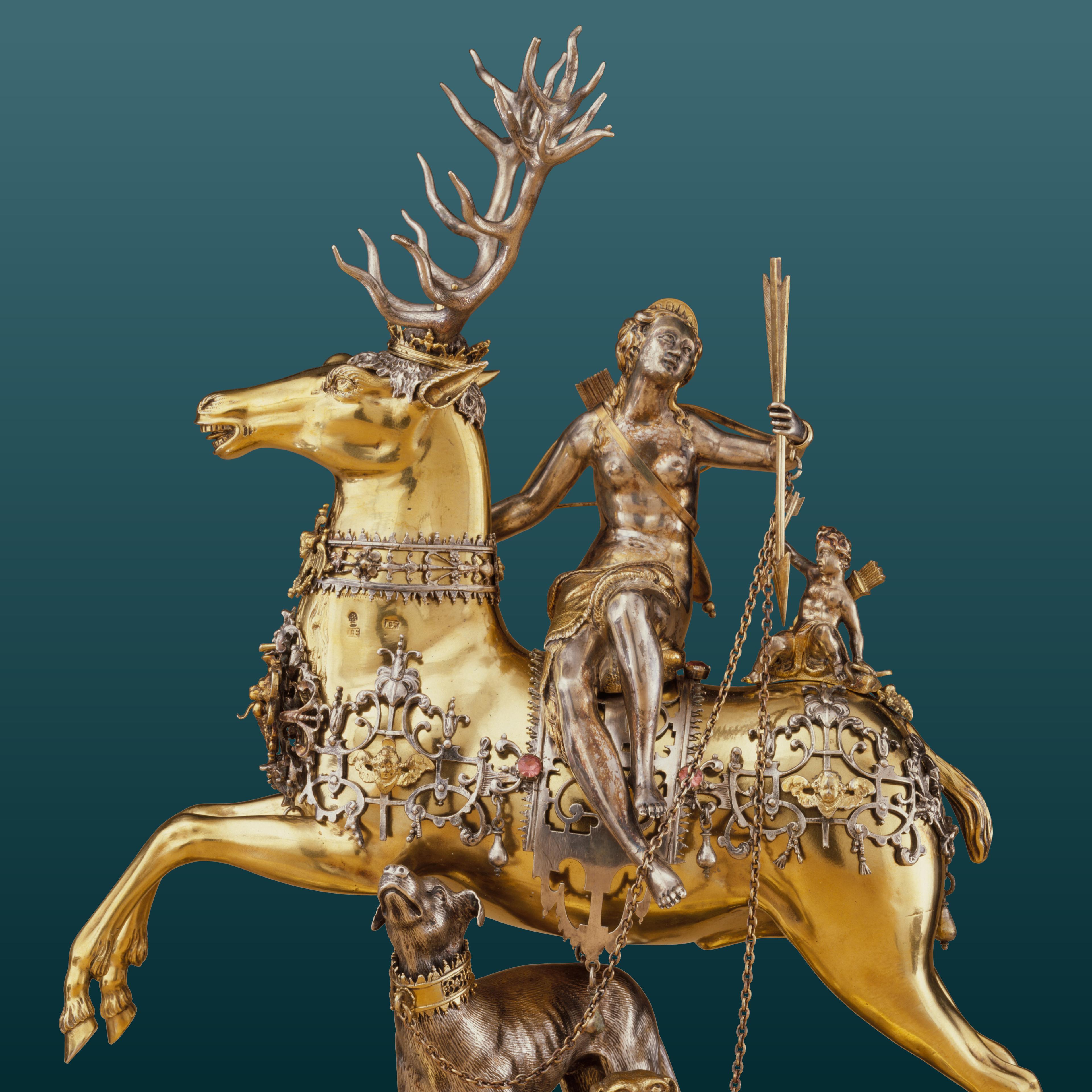This close-up photograph showcases an intricate gold statue of an antlered horse, featuring a mix of ornate materials including gold and bronze. The horse is dynamically poised in mid-buck and is adorned with elaborate jewelry that includes an ornate choker around its neck and decorative accessories along its back and front. A majestic crown sits at the base of the horse's tall, silver antlers. 

On the horse's back is a cherub, poised with arrows in its right hand and an arrow sling visible over its shoulder. The cherub's left hand grips the side of the horse for balance. A second, smaller cherub is seated on the horse's hindquarters, also equipped with a sling of arrows. Beneath the horse, a bronze dog with a matching ornamental choker gazes upwards towards the majestic creature and its riders. The entire statue presents an eye-catching blend of detailed craftsmanship and dynamic composition set against an aquamarine-colored background.